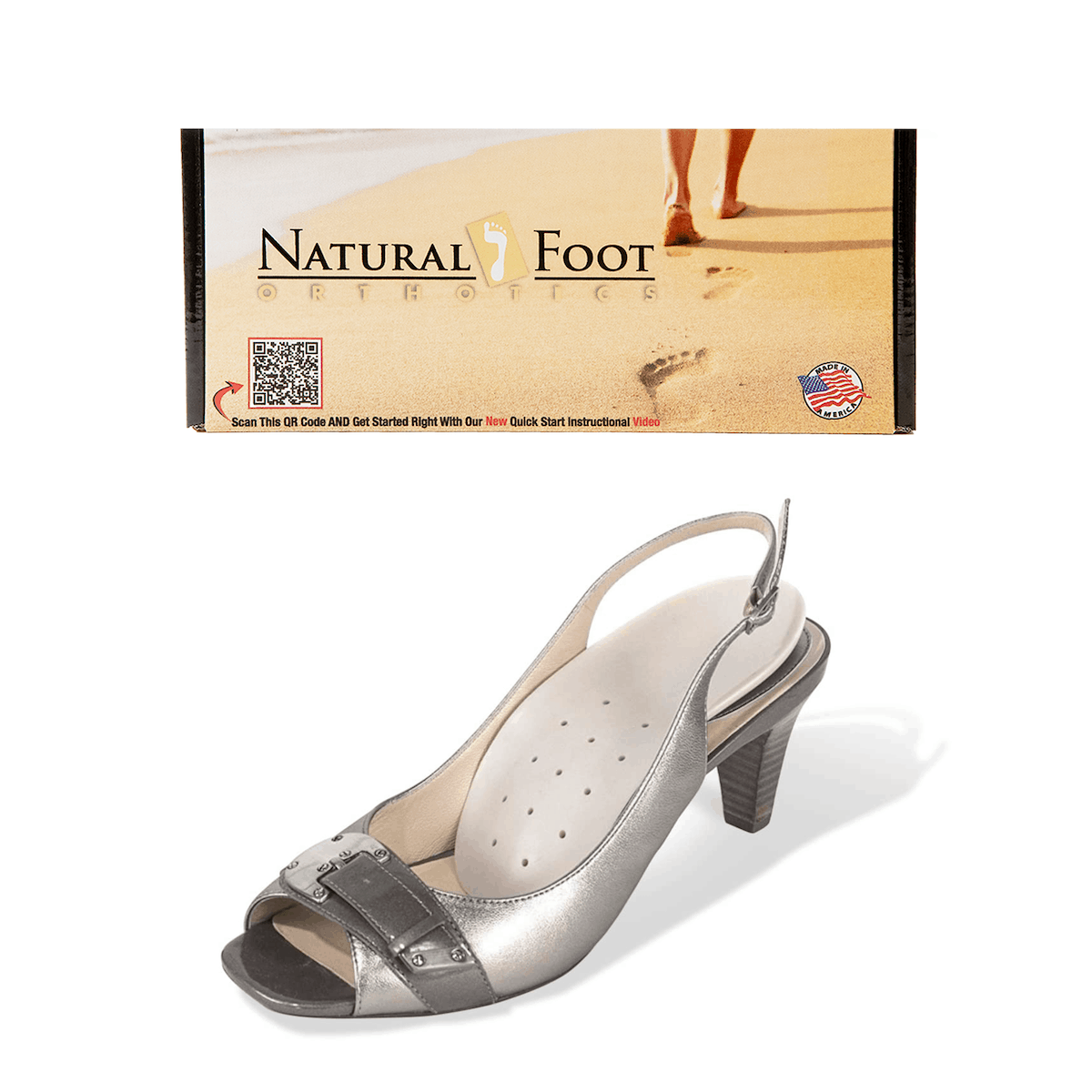The image depicts a stylish open-toed, slingback kitten heel shoe in silver and gray, featuring a metallic buckle on the instep and heel strap. The shoe also boasts a white cushioned footpad with air holes on the sole. Positioned beneath a rectangular advertisement, the ad prominently displays the text "Natural Foot Orthopedics" against a background image of sandy beach footprints and a person's legs up to the shins, seemingly walking away. On the bottom left corner of the ad, there is a black and white QR code with a prompt to scan for a quick start instructional video. In the bottom right corner, the ad features an American flag symbol with the caption "Made in America."